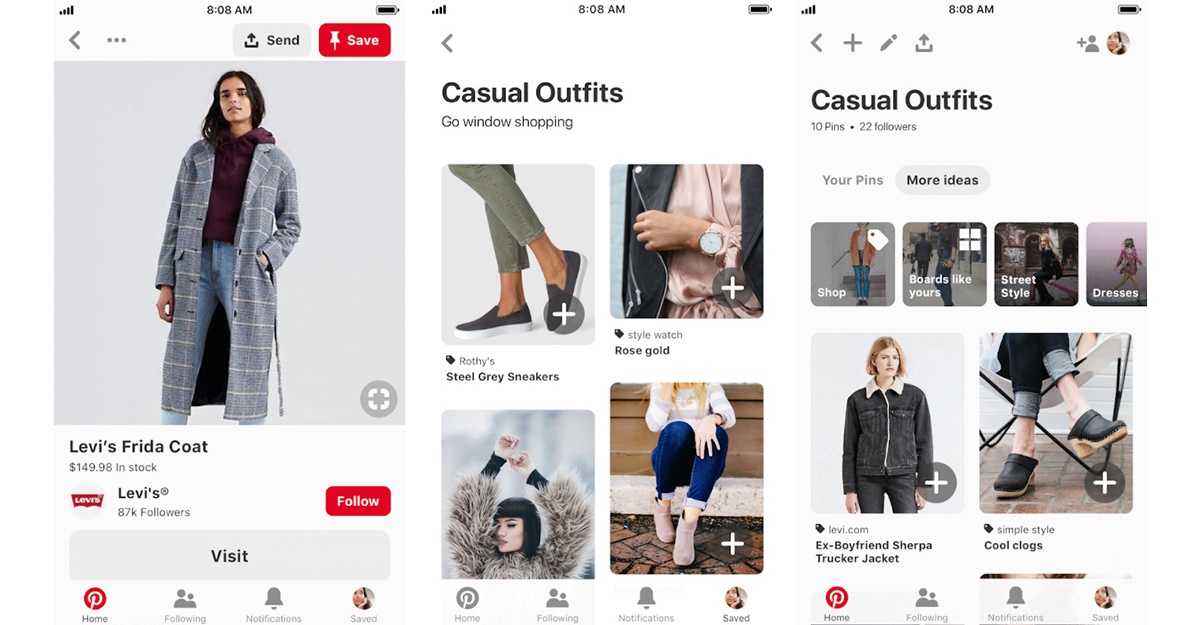Here is a cleaned-up and detailed caption for the series of screenshots from the Pinterest mobile app:

---

The image depicts three side-by-side screenshots from the Pinterest mobile app. 

1. **Left Screenshot**:
   - Features a large photograph of a model wearing Levi's Frida Coat.
   - Below the image, "Levi's Frida Coat" is displayed in bold black letters along with the price and availability status ("in stock").
   - The Levi's profile icon is visible on the bottom left corner, accompanied by "Levi's" text and the follower count of 87,000.
   - A red "Follow" button is located on the far right, and below this, a large gray "Visit" button is prominently displayed.

2. **Middle Screenshot**:
   - Showcases the "Casual Outfits" page, with the title "Casual Outfits" in large black bold print at the top.
   - Subheading "Go window shopping" appears in smaller gray print beneath the title.
   - The page features four thumbnail images, each depicting different outfit inspirations, with a plus icon in the bottom right corner of every image.

3. **Right Screenshot**:
   - Displays another "Casual Outfits" page, this time highlighting the number of pins and followers of a personal board named "Casual Outfits."
   - Subsections such as "Your Pins" and "More Ideas" are listed, with "More Ideas" highlighted.
   - Four horizontal thumbnail categories are displayed: "Shop," "Boards like yours," "Street Style," and the partially cropped out "Dresses."
   - At the bottom, there are two larger pins featuring a jacket and a pair of shoes, respectively.